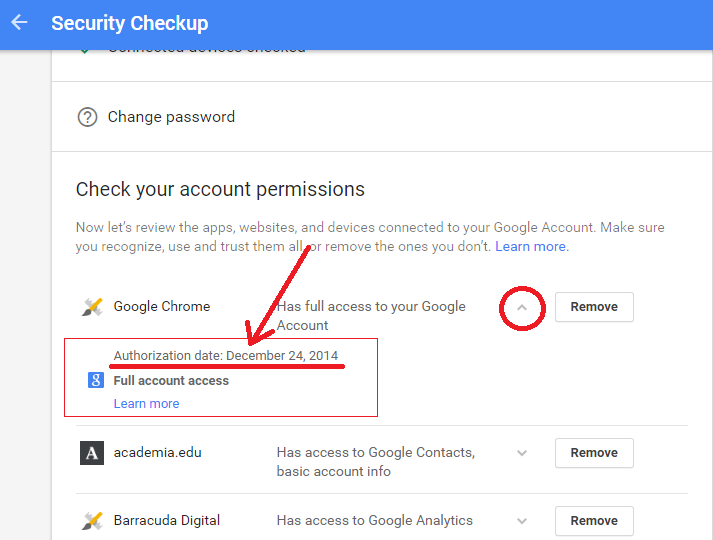The image depicts a website conducting a security checkup for a Google account. At the top, a blue progress bar spans horizontally across the screen. To the left of the bar, an arrow points left, suggesting the possibility to return to a previous step.

Below the blue bar, there's an obscured white section, partially covered by the blue bar, making the text unreadable. The next section, also in white, prominently features a "Change Password" option next to a small circle with a question mark inside it, possibly indicating help or more information.

Further down, the screen displays a prompt urging users to "Check your account permissions." It includes a detailed message: "Now let's review the apps, websites, and devices connected to your Google account. Make sure you recognize, use, and trust them all or remove the ones you don't." Within this message, the phrase "Learn more" appears in blue text, likely serving as a hyperlink for additional information.

An arrow extends from the "all or remove" section downwards, directing attention to a red-outlined box. This box highlights the "Authorization date: December 24, 2014," underlined in red to emphasize its importance. A red arrow points towards this date, and a similarly colored circle surrounds an "arrow up" button next to the "Remove" button, both designed to manage account permissions.

Additionally, two other categories, "Academia.edu" and "Barracuda Digital," are listed below. Each entry indicates these services have access to the Google account and provides options to remove them if they are no longer needed or trusted.